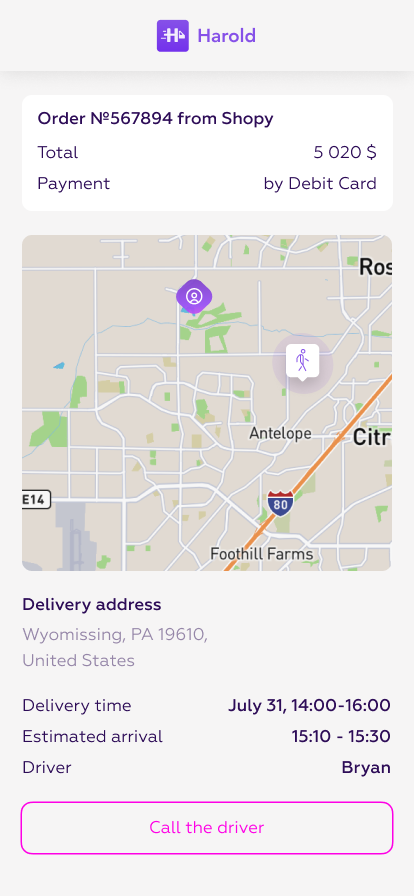This image is a screen capture from a mobile device display of an app, shown in portrait orientation. The app title, "Harold," is prominently displayed at the top of the screen in purple text, accompanied by a logo on the left—a purple square featuring a stylized light gray "H." The overall color scheme of the app consists of white, gray, black, and purple.

The primary content of the screen features a light gray background with a centered square map application reminiscent of Google Maps. The map itself is primarily gray with white road delineations, including a significant orange highway, Interstate 80, which cuts diagonally across the lower right-hand corner. Specific locations such as "Antelope" and "Foothill Farms" are labeled. A prominent purple icon marks a specific location on the map.

Below the map, the delivery address is displayed: "Wyomissing, PA 19610, United States." Additional delivery information follows, including delivery time, estimated arrival, and driver details. At the very bottom of the screen, there is a pink-outlined button labeled "Call the Driver."

Just above the map, there is further order information detailing the order number, total amount, and the payment method used.